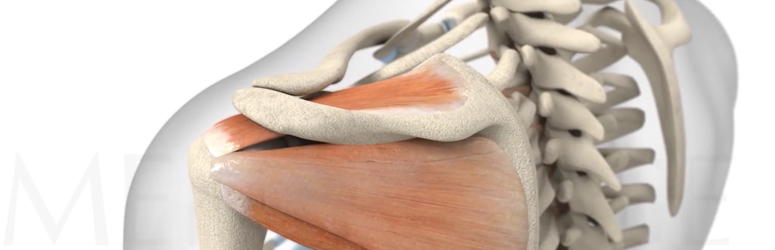This detailed anatomical image, rectangular and horizontally oriented, resembles an illustration from a science or medical book. It offers a rear view of the upper back, focusing on the left shoulder and part of the spine. The image showcases a transparent figure, revealing a meticulous depiction of bones, muscles, tendons, and ligaments. Prominently visible are the white bones of the backbone or spine, extending from the neck down to the mid-back, and the left scapula. The left shoulder muscle is vividly illustrated in shades of reddish-orange, highlighting the rotator cuff and labrum. The right shoulder and rib cage are partly visible, though the right-side muscles are absent. The left arm begins to emerge from beneath the tendons and ligaments but is truncated before the elbow. This detailed image, utilizing distinct color differentiation (off-white bones and reddish-orange ligaments), is ideal for educational purposes, helping students or patients visualize the intricacies of human anatomy and potential injuries.